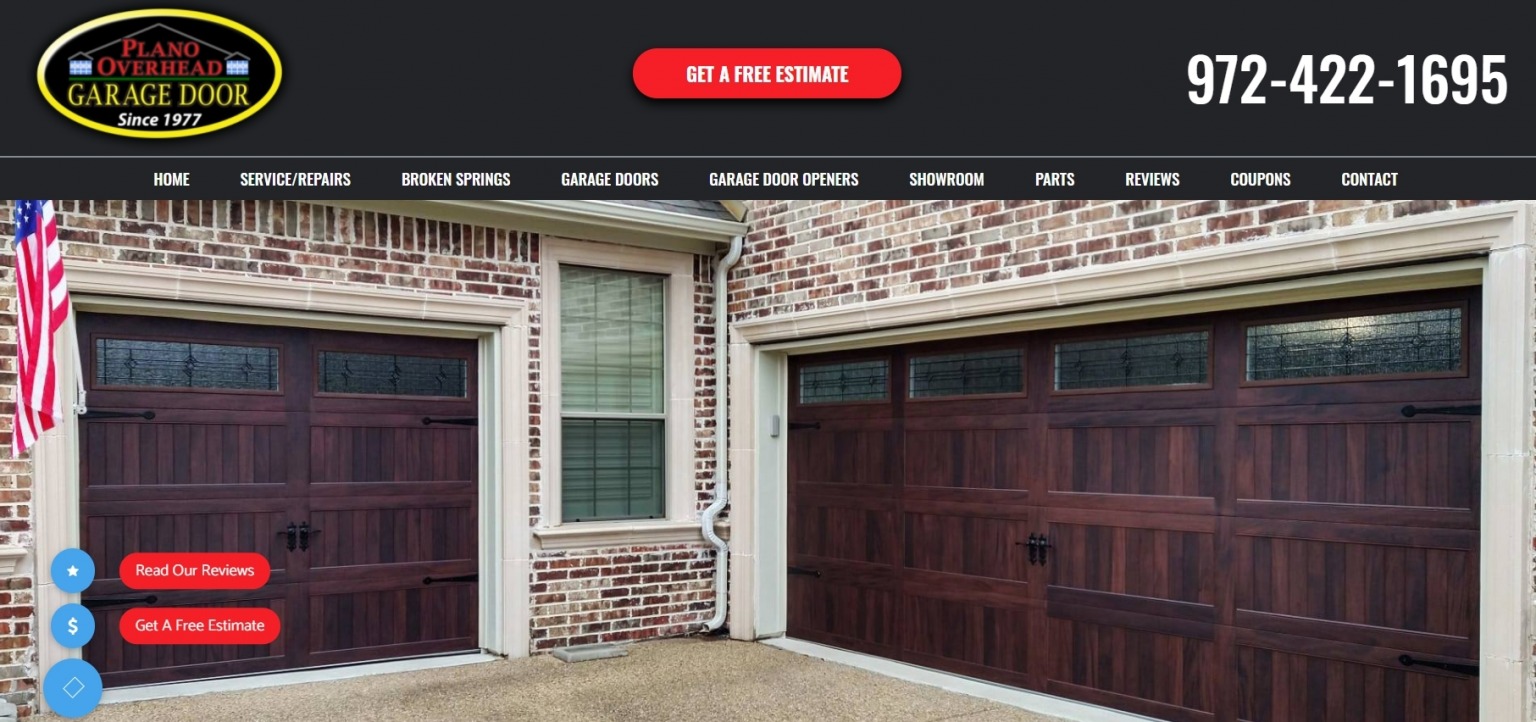The image depicts the homepage of a website for a garage door store named "PLANO Overhead Garage Door," established in 1977. The logo is prominently displayed, featuring "PLANO Overhead" in red, "Garage Door" in gold, and "Since 1977" in white, all set against a black background and circled by a yellow oval. 

At the top center of the page, there is a red button with white text that reads "Get a Free Estimate." On the right side, the phone number "972-422-1695" is displayed in the largest font on the page, also in white.

Below the logo, a white navigation menu on a black background lists various options: "Home," "Service/Repairs," "Broken Springs," "Garage Door," "Garage Door Openers," "Showroom," "Parts," "Reviews," "Coupons," and "Contact."

Further down, there is an image of a home with two garage doors; the larger one is to the right, and the smaller one is on the left. Both doors are made of dark brown wood with visible grain. To the left of the image are two red buttons labeled "Read Our Reviews" and "Get a Free Estimate." Additionally, there are three blue round icons featuring a star, a dollar sign, and a square, respectively.